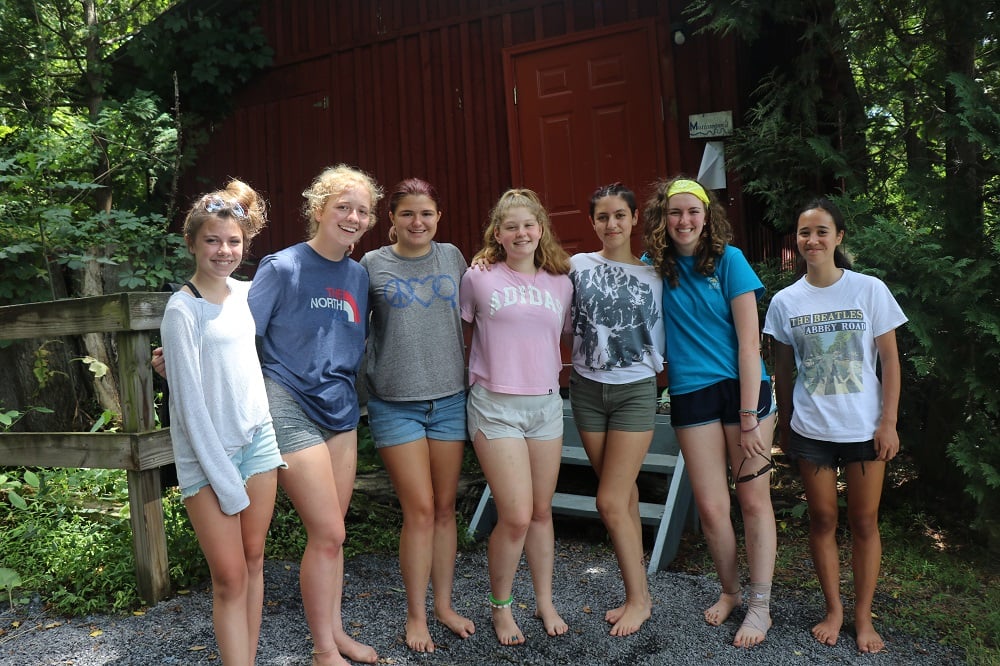In this photograph, seven young barefoot women are posing happily in front of a small red corrugated metal cabin, which features a single red six-paneled door and gray wooden steps. The group stands on a bed of gray gravel, with lush green shrubbery and a sunlit forest in the background. Starting from the left, the first girl is wearing short denim cut-off shorts, a long-sleeve white shirt over a black tank top, and has her hair pulled into a ponytail on the left side of her head. Next to her, a girl in gray shorts sports a blue short-sleeve shirt with "The North" printed on the front. The third girl wears blue denim shorts and a gray short-sleeve shirt adorned with a blue peace sign, heart, and magnifying glass. In white shorts and a pink short-sleeve shirt with "Adidas" in white text, the fourth girl stands smiling. The fifth girl showcases green denim shorts paired with a white graphic shirt featuring the outline of a white deer in a forest. There’s a variety of hair colors among them, including curly long brown, black tied back, blonde, and vibrant burgundy red. They stand close together, with arms around each other's shoulders, indicative of a joyful summer camp memory.